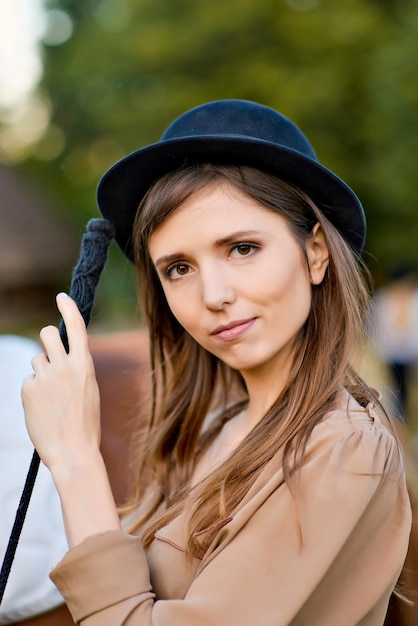The photograph portrays a young woman, likely in her 20s, with a light complexion, dark brown eyes, and long brunette hair hanging down on both sides. She wears a brown long-sleeved shirt and a dark hat, possibly a fedora, although some may describe it as a dark blue felt hat. The image is a close-up, taken outdoors during the daytime with a blurred background showing hints of green trees. She holds a long, thin navy blue object, potentially a whip or a cane, in her left hand, raising it near her face. Her right arm is not visible in the photo. The woman is looking directly at the camera with her head tilted slightly to her right, and has a subtle smirk on her face. Overall, the photo gives an impression of an equestrian theme, as suggested by her attire and the presence of the whip.